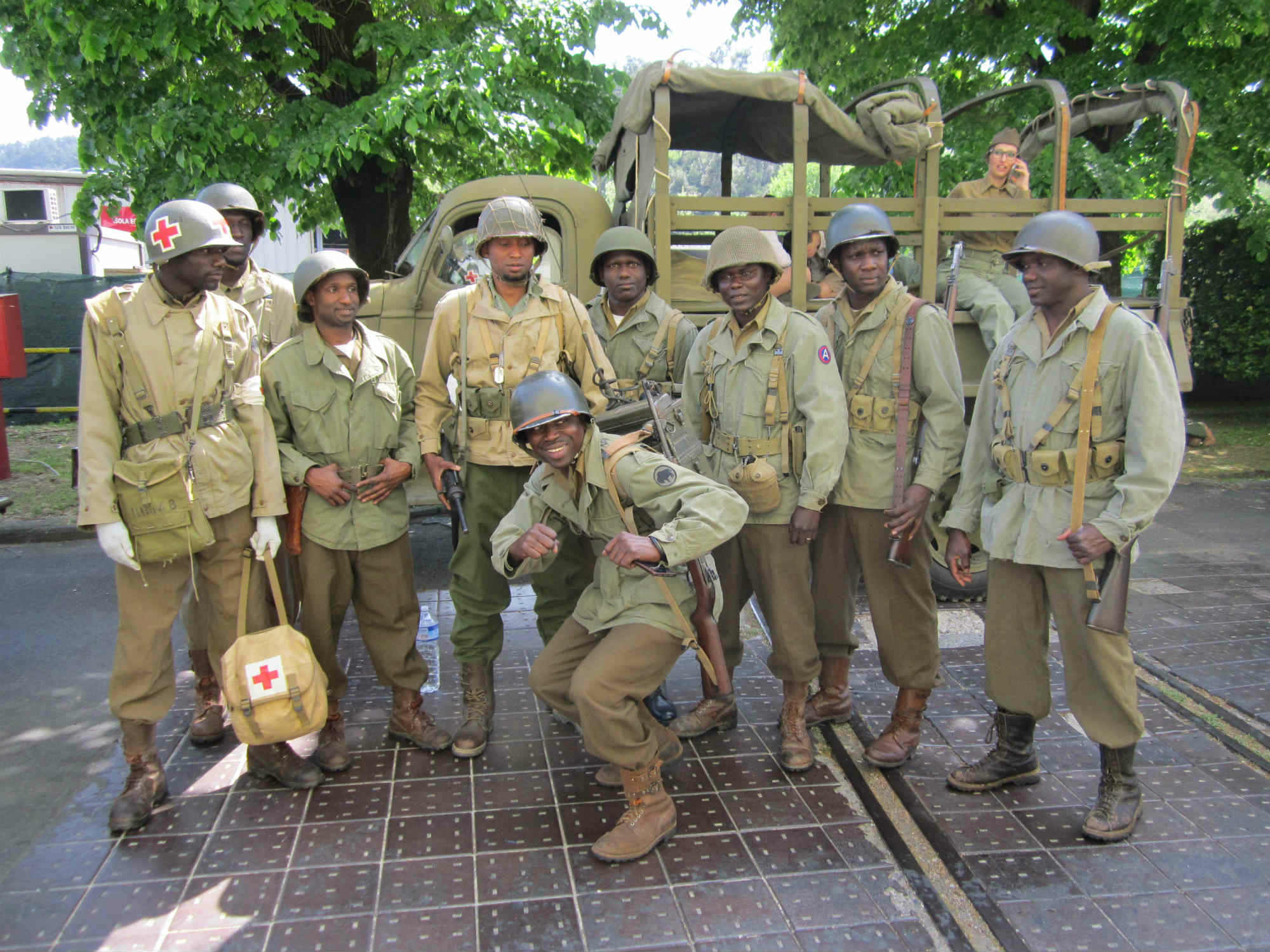The image is a detailed color landscape photograph featuring a group of nine black soldiers dressed in an assortment of military uniforms and helmets. They are standing in a semi-circle, with one soldier in the center slightly crouching and smiling. The other soldiers, though not all smiling, are looking in various directions. The uniforms are a mix of light green, yellow, and different shades of boots, suggesting historical or reenactment attire, possibly from the World War II era. One soldier on the far left is holding a backpack with a white background and a red cross, a symbol also present on his helmet, indicating he is a medic. In the background, there is a green military troop transport truck with a tarpaulin rolled back. Inside the truck, a white woman, dressed similarly to the soldiers but with cat-eye shaped vintage glasses and a cloth hat, is talking on a cell phone, hinting at a possible reenactment setting. They are standing on a corrugated metal platform with brown tiles and yellow stripes outlined in black. The backdrop includes partial views of a tree with green foliage and distant buildings obscured by the standing soldiers.